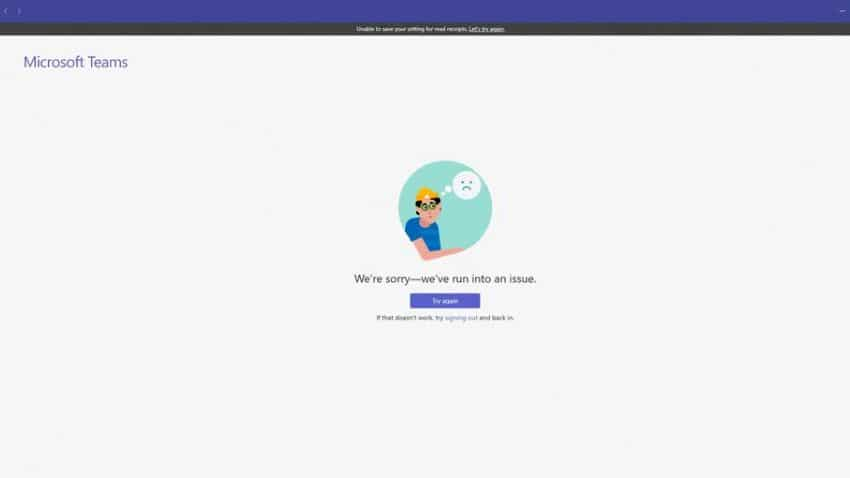This screenshot from Microsoft Teams captures an error message interface. At the very top, there's a deep blue navigation bar, followed by a slightly smaller black bar. Although the text on the black bar is semi-pixelated and difficult to read, it appears to convey an error message along the lines of "unable to save your changes," with the phrase "let's try again" underlined in white, suggesting that it is a clickable link to retry the action.

In the main section of the screenshot, a large gray box dominates the screen, representing the default user interface of Microsoft Teams. Centered within this box is an illustration of a man wearing a yellow construction hat and glasses, dressed in a blue shirt, with his arm resting inside a circle. A thought bubble emanates from his head, leading into a frowny face, visually expressing dissatisfaction or a problem.

Below this image, there's a message stating, "We're sorry – we've run into an issue." Directly under this text is a prominent blue button labeled "Try again," inviting users to attempt the operation once more. Further down, additional instructions suggest, "If that doesn't work, try signing out and back in," with the term "signing out" highlighted in blue, indicating it is a clickable link for users to follow this troubleshooting step.